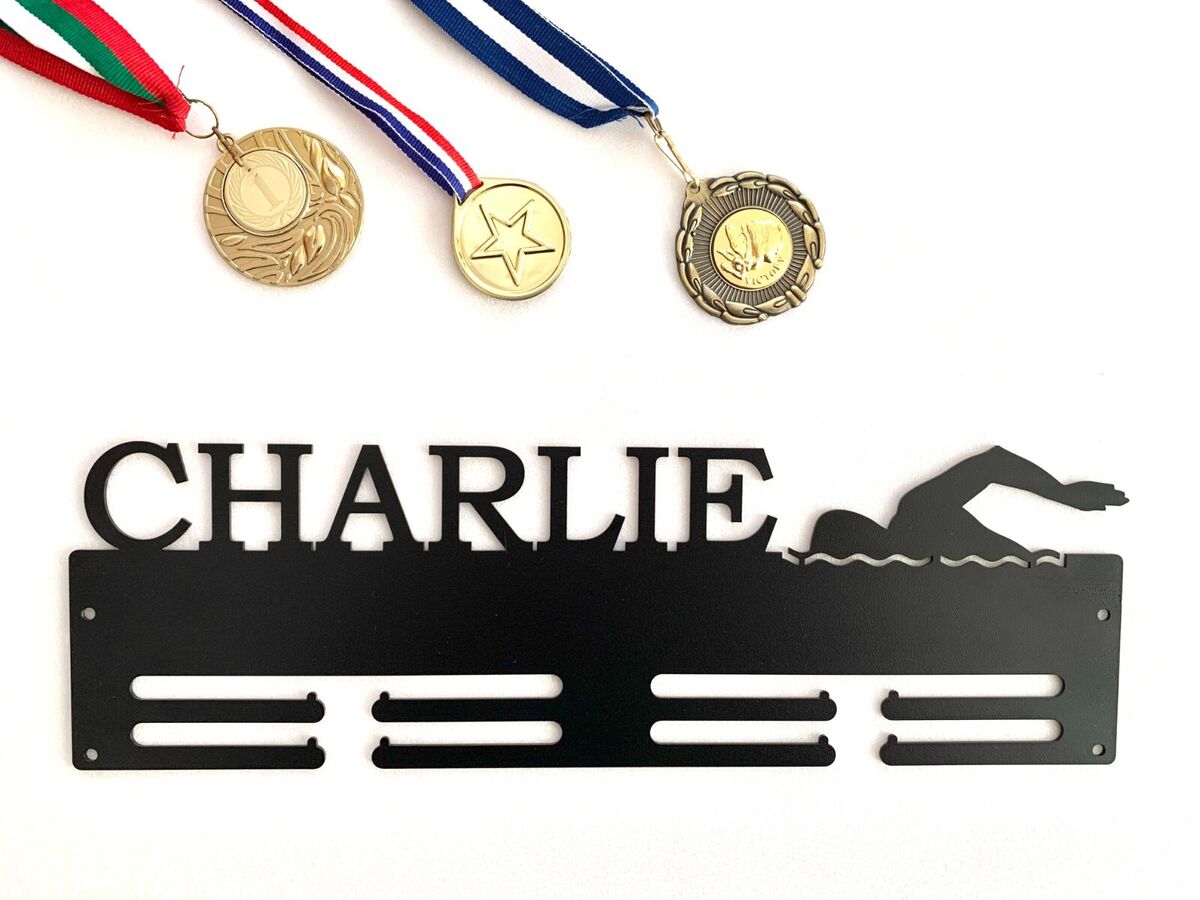The image showcases a rectangular black plaque, likely meant to be hung on a wall, prominently featuring a cutout silhouette of a swimmer with one arm extended above the water, complete with wave-like ripple lines beneath. To the left of the swimmer, the name "Charlie" is inscribed in bold black letters. The bottom part of the plaque has cutouts that resemble slots or spaces, suggesting either a decorative element or a functional design, with small holes on either side possibly meant for mounting.

Above this plaque, three medals, each distinct in design and shape, are arranged diagonally from the upper left corner of the image. The ribbons of the medals extend out of the frame, but the medals themselves are clearly visible in the upper center of the image. 

The leftmost medal, attached to a dark red and green lanyard, is gold and features a larger circular design with intricate leaves and wave patterns, containing a smaller medallion inscribed with the number "1" at its center. 

The middle medal, hanging from a blue, white, and red lanyard, is also gold and showcases an embossed star within its circular form. 

The rightmost medal is affixed to a blue lanyard with a fine white stripe. This medal has a bronze leaf-patterned border with a gold center that appears to bear the word "Victory," surrounded by additional circular detailing. All of this is set against a plain white background, emphasizing the detailed craftsmanship and significance of each element.